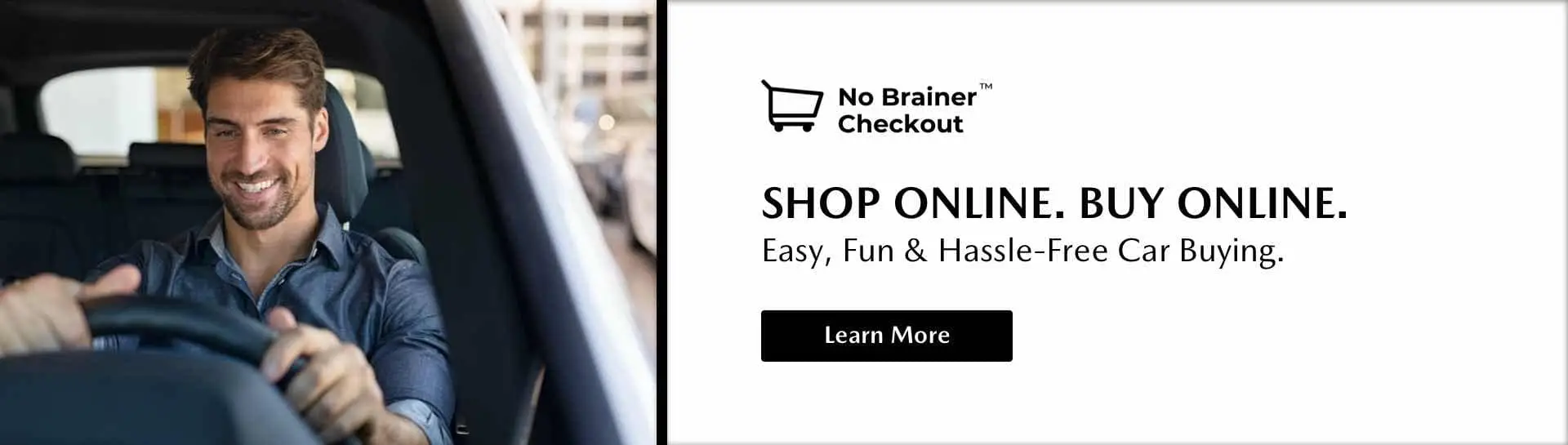This digital advertisement features a well-dressed Caucasian man seated in the driver's seat of his car, prominently positioned on the left side of the ad. With brown hair and a slightly unkempt 5 o'clock shadow, he is smiling broadly, exuding a sense of contentment. His hands are positioned firmly at the 10 and 2 o'clock positions on the steering wheel, adhering to traditional driving posture. The man wears a collared, three-button down shirt, and the car's interior is sleek and black. Though the exact color of the vehicle is unclear, the background shows a hint of traffic in the distance, contributing to the context of his location.

On the right side of the advertisement, bold text reads "No Brainer Checkout" above an illustration of a shopping cart. Below this, the message "Shop Online, Buy Online – Easy, Fun, and Hassle-Free Car Buying" is prominently displayed, occupying approximately 60% of the ad space. To finalize the call-to-action, a "Learn More" button is included at the bottom. The background of the text section is white, ensuring that the promotional message stands out sharply against the rest of the content. This rectangular ad effectively merges visual and textual elements to create a compelling narrative about convenient and enjoyable car buying.